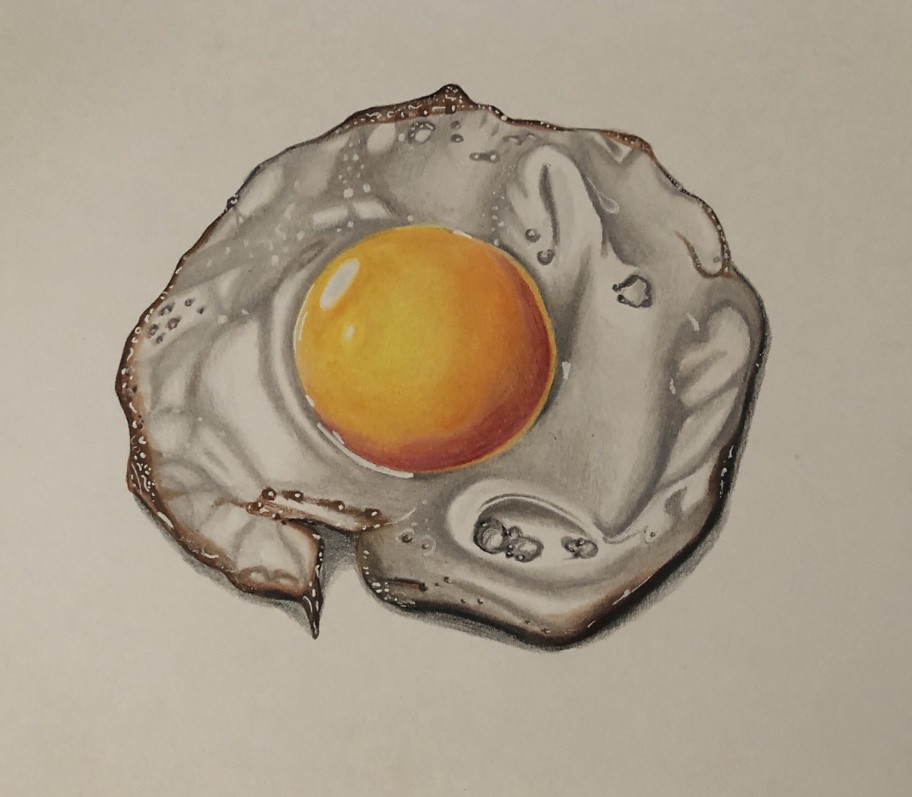This is a square-shaped, stylized artistic illustration of a fried or soft-boiled egg, most likely created digitally. The image is set against an off-white or beige background, which gives it a slightly darker appearance than a pure white backdrop would. The egg is perfectly centered, highlighting its almost surreal perfection.

The egg features a flawlessly round yellow yolk with a light glinting off of it, suggesting a solid, unbroken yolk. Encircling the yolk is the translucent egg white, which exhibits a range of colors—gray, yellow, and white—with hints of crispiness at its edges. This crispiness is marked by browned areas with tiny, bubble-like holes and indentations, indicating where the egg white has browned and crisped perfectly. The outer lit circle of the egg white also contains small, bubble-like textures, adding to the detailed realism of the illustration. There is no signature on the artwork, further emphasizing its digitally rendered, photorealistic nature.